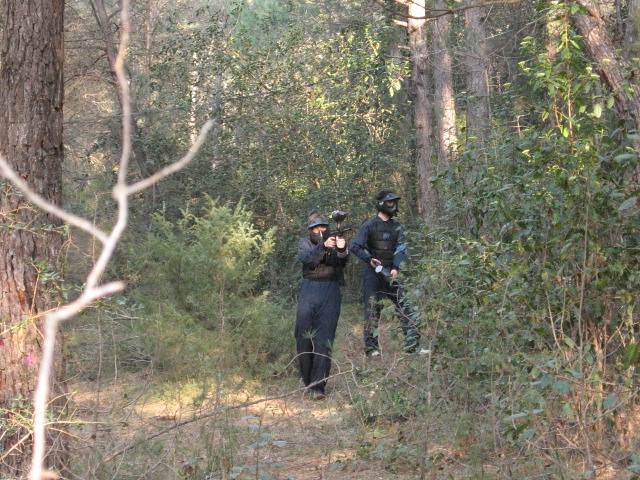In a densely wooded area illuminated by the last slivers of evening sunlight, two paintball fighters navigate a narrow, rustic path that's simply a mowed-out section of the forest floor. Clad in dark clothing for camouflage and wearing protective vests and full-face masks for safety, they are fully equipped for the game. Their compressed air guns, designed to shoot paint pellets, are at the ready. One fighter, on the left, is actively pointing and aiming at a target, while the other stands vigilantly behind trees, observing the scene. The interplay of light through the foliage casts a dramatic ambiance over the tense, strategic moment in their paintball match.